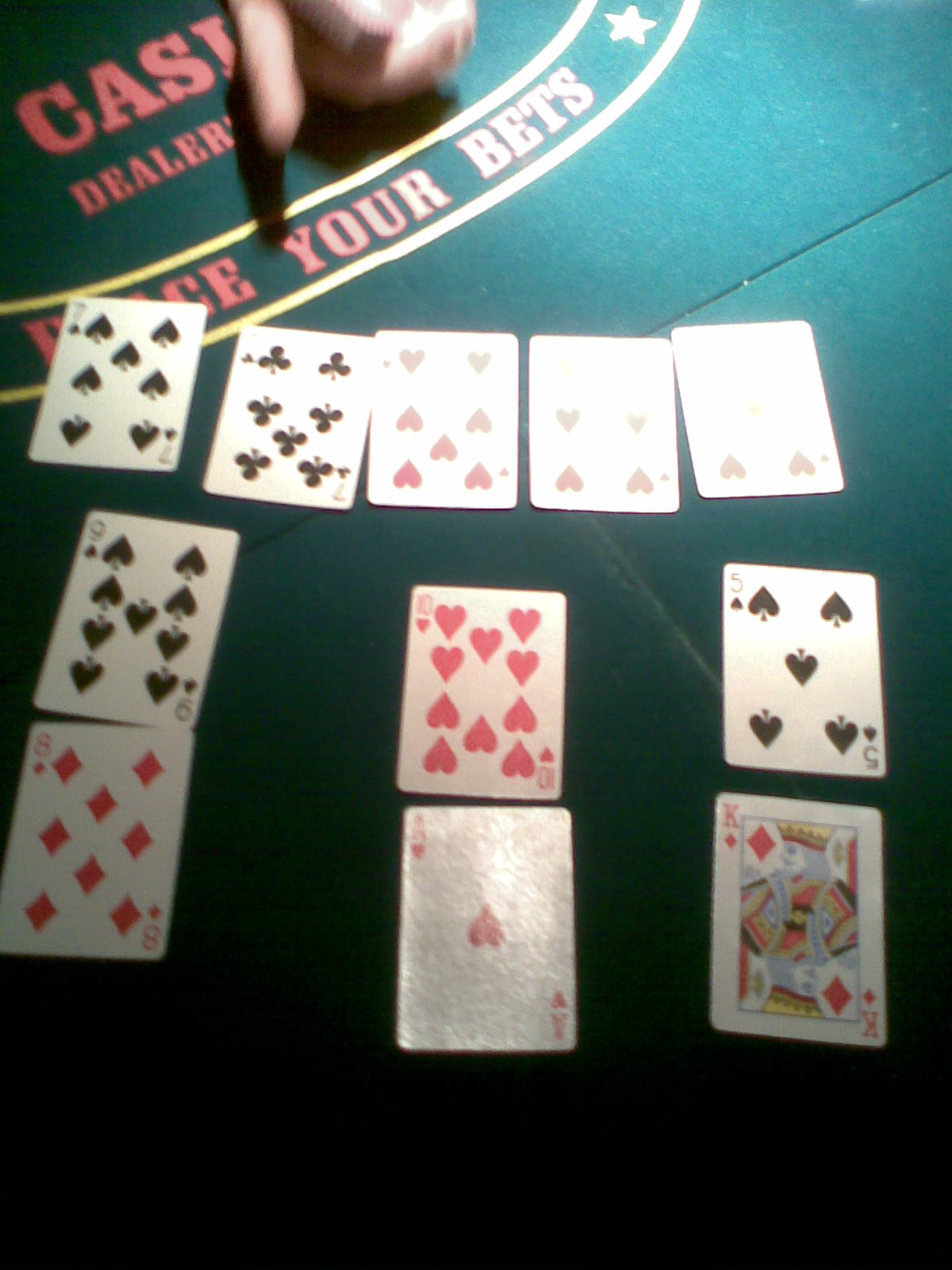The image depicts a casino dealer's table in a blurry color photograph taken in portrait orientation. The setting appears to be dimly lit, with the table's dark surface—possibly black or dark green—serving as the background. A hand extends from the top edge of the photo, pointing towards the table. 

At the upper center of the image, partially visible red lettering spells out "CASINO" with "DEALER" written beneath it in smaller white text. Below this, a yellow-outlined ribbon or banner displays the phrase "PLACE YOUR BETS" with a small star accentuating the design.

Central to the image is a spread of five face-up cards arranged in a row, though they are noticeably reflective. The identifiable cards include the Seven of Spades, Seven of Clubs, and Seven of Hearts. The fourth and fifth cards are obscured by glare but seem to be heart-suited cards as well.

Below this row, there are three columns, each containing two cards. The left column reveals a Nine of Spades above an Eight of Diamonds. The middle column shows a Ten of Hearts positioned above an Ace of Hearts, marred by significant glare. The third column features a Five of Spades with a King of Diamonds beneath it.

The overall atmosphere is one of engagement and anticipation, capturing the essence of a bustling casino environment dedicated to the thrill of gambling.